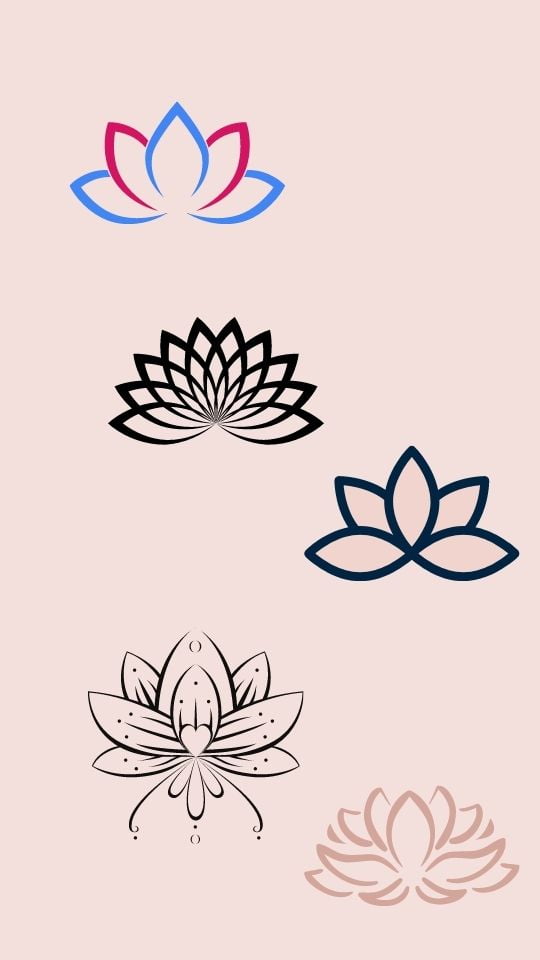This image features a collection of graphic design-style floral illustrations against a beige, slightly peach or pinkish background. The flowers are depicted with distinct, pointy petals oriented upwards. Starting from the top left, the first flower showcases three blue petals surrounded by two red ones. Adjacent to it is another flower composed entirely of black petals, intricately interconnected. Further down, there is a flower with five petals outlined in blue. Towards the bottom left, a more ornate design emerges, featuring black lines and small black dots around the flower, and additional detailing below it, with a heart-like shape at its center. Finally, in the bottom right corner, there's a flower with more petals drawn with a dark beige or brown outline. Each flower possesses unique characteristics, contributing to a rich tapestry of illustrative floral art.